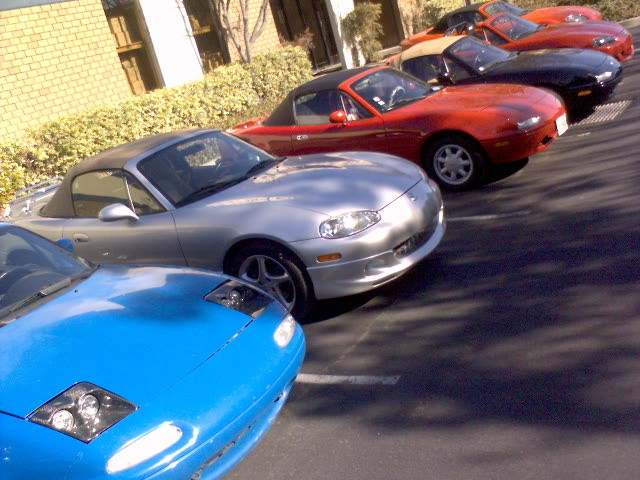The color photograph depicts a parking lot with six sleek sports cars, all backed into their parking spaces. The cars are lined up from the bottom left corner as follows: a bright sky blue convertible, a silver car, a red convertible, a black convertible, a burgundy car, and another red convertible in the distance. Notably, the majority of these convertibles feature black drop tops, except the black car, which has a tan drop top, and the distant red car, which also has a black drop top. They are parked against the backdrop of a fading yellow brick building adorned with a row of bushes. The building features several windows, and the parking lot's white lines clearly delineate the individual spaces. Shadows from an off-screen tree stretch across the blacktop, adding depth to the scene.